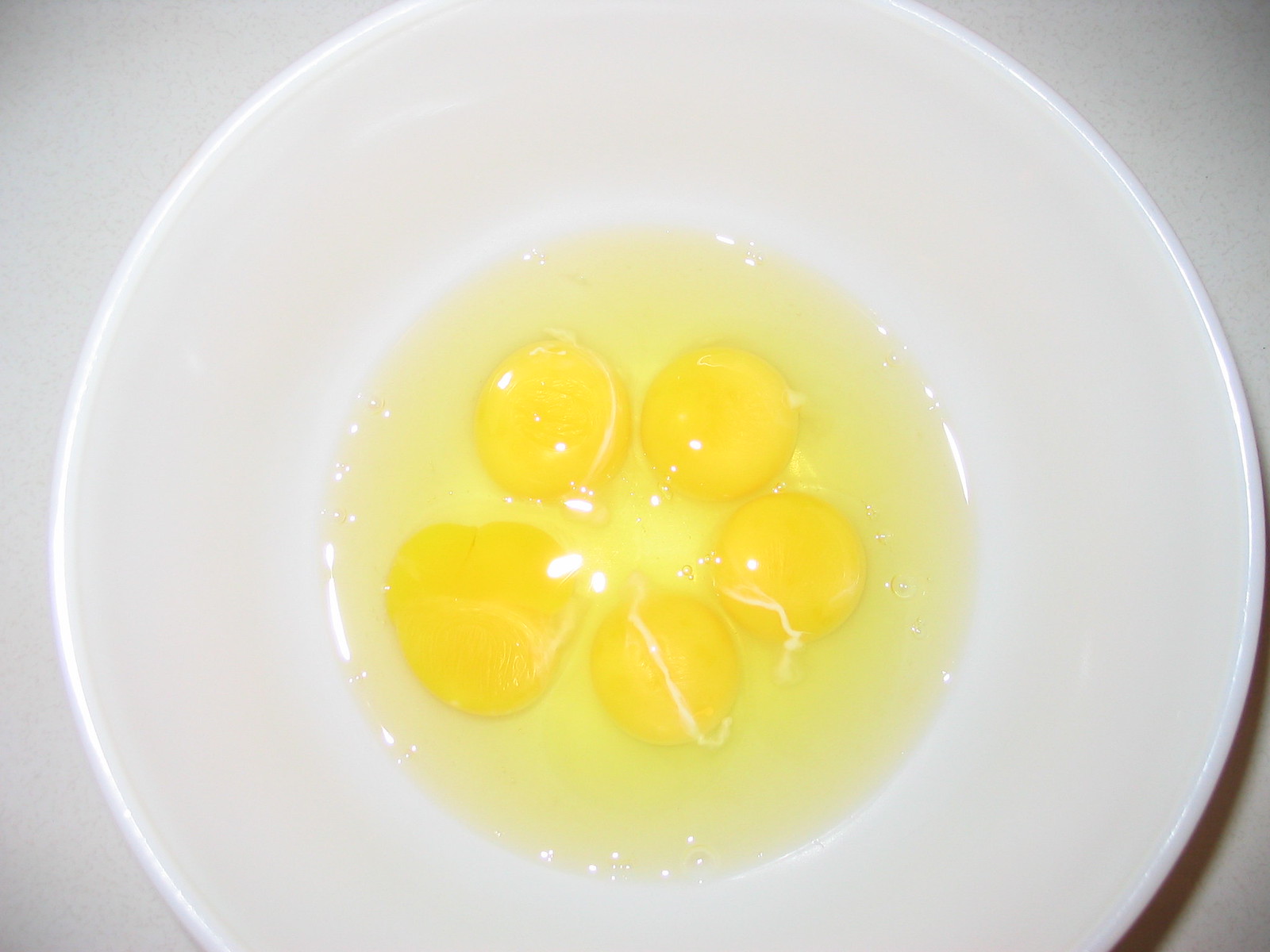This overhead color photograph captures a high-sided white mixing bowl placed on a light gray surface, containing five cracked chicken eggs. Four eggs display their intact yellow yolks, while the yolk on the lower left is broken but not yet stirred. The albumen, or egg white, remains undisturbed around the yolks. The composition suggests that the eggs are prepared for making an omelet or scrambled eggs. The soft lighting highlights the subtle details in the yolks and the bowl, enhancing the overall clarity and texture in the image. The bowl's placement and the contents give a clear sense of the beginning stages of a cooking process.